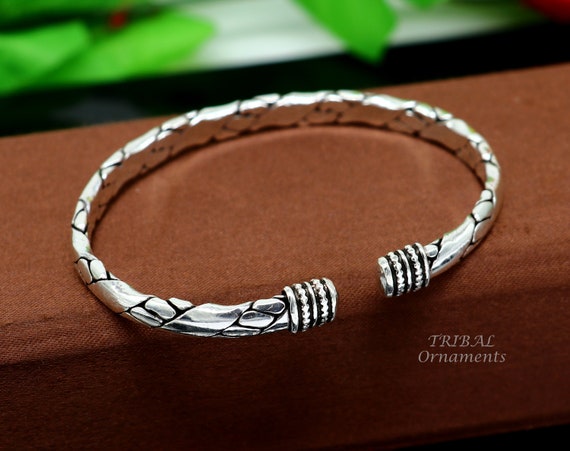The image features an intricately designed wristband, resembling a thick metallic ring crafted from a silverish material. The wristband is adorned with a unique pattern where silver segments are interspersed with black grout-like textures, creating an oblong shape throughout the design. The clasp, prominently displayed towards the camera, showcases an alternating pattern of silver and black rings, highlighting the intricate craftsmanship. The wristband rests on a reddish-brown cloth, adding a rustic backdrop that complements the metallic hues. The background is a mix of dark green foliage, with vibrant green leaves subtly peeking through, creating a natural and earthy environment. In the bottom right corner, a watermark reading "Tribal Ornaments" subtly identifies the origin or brand of the jewelry.